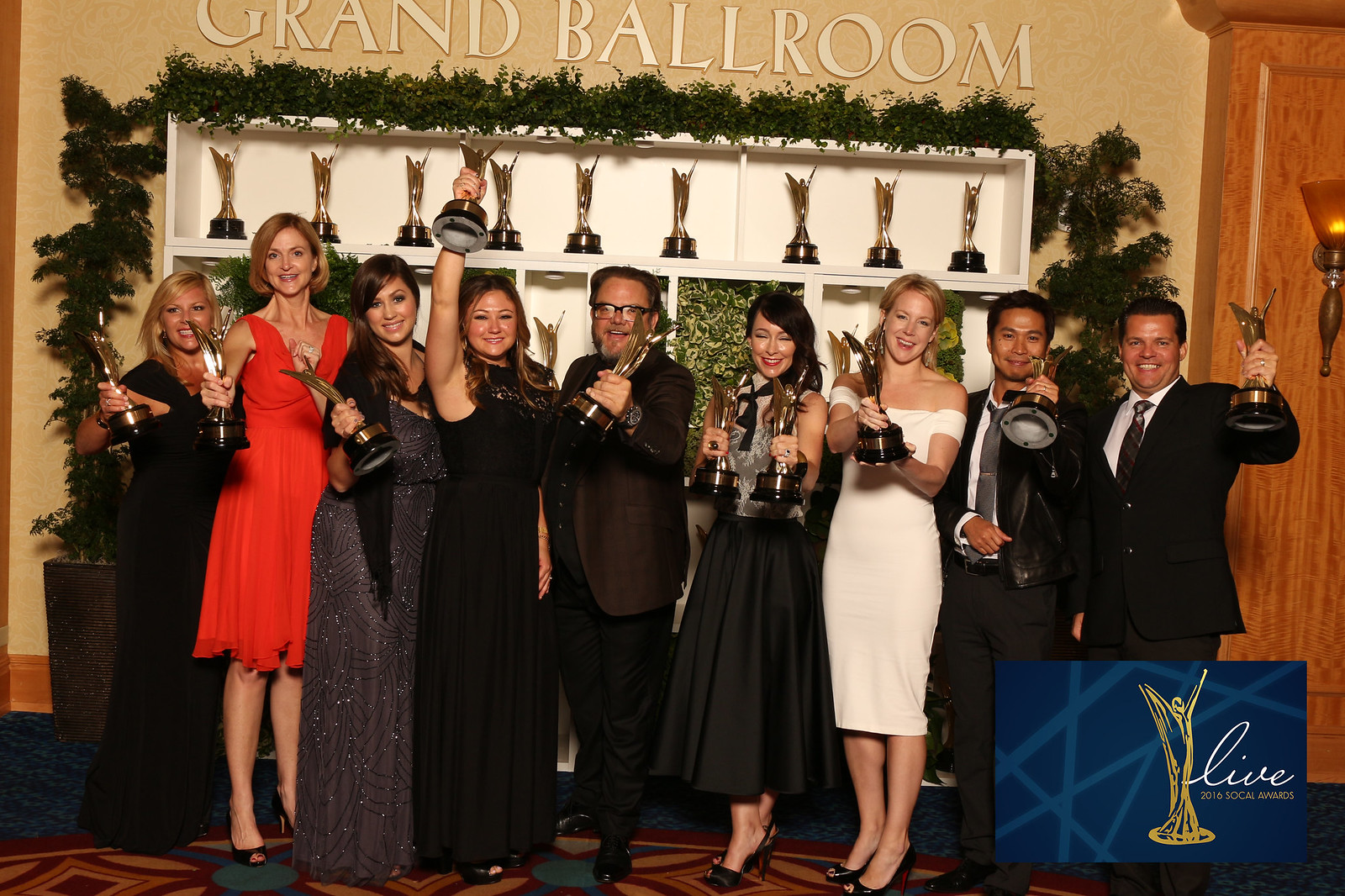In this image, a group of nine people is standing proudly with their trophies at what appears to be an award ceremony. The background features a beige-tan wall with the inscription "Grand Ballroom" in white, outlined in brown at the top. To the right side, there's a wooden pillar adorned with a wall lamp. Additionally, it has blue and white emblem in the bottom right corner, depicting a trophy with angel wings and an arm raised victoriously, accompanied by cursive writing.

The scene is well-illuminated, showing a white trophy case behind the group, containing nine trophies that resemble the emblem. Draped over the case is a festive, green leaf garland, adding a touch of celebration to the setting.

From left to right, the nine award recipients are:
1. A woman in black with blonde hair, holding her trophy in her right hand.
2. A taller woman in a red sleeveless dress with shorter hair, also holding her trophy in her right hand.
3. A woman in a black evening gown with long hair, holding her trophy aloft.
4. A woman in a black dress with brown hair, lifting her trophy above her head.
5. A man with short hair, glasses, and a black suit, clutching his trophy with his left hand.
6. A woman in a black dress holding two trophies, one in each hand, with her eyes closed.
7. A woman in an off-the-shoulder white knee-length dress, holding her trophy with both hands.
8. A man in a black suit with an open jacket, grey tie, and white shirt, holding his trophy in his left hand.
9. A man, smiling proudly, in a black suit with a black tie and white shirt, holds his trophy up with his left hand.

They stand on a carpeted floor with a darker section behind them, embodying a sense of accomplishment and celebration at this award ceremony, likely the 2016 SoCal Awards as indicated by the emblem.